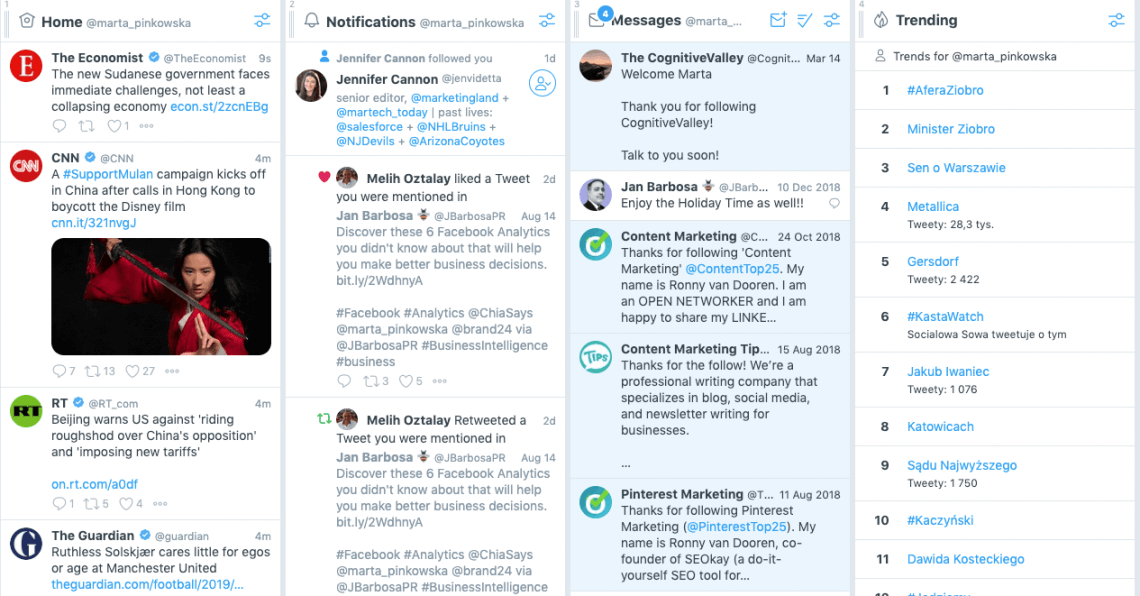In this image, the Twitter app displays several news updates from prominent media outlets alongside trending topics. The news messages include:

1. **The Economist:** "The new Sudanese government faces immediate challenges, not least a collapsing economy."
2. **CNN:** "A support Mulan campaign kicks off in China after calls in Hong Kong to boycott the Disney film."
3. **Reuters:** "Beijing warns the US against riding roughshod over China's opposition and imposing new tariffs."
4. **The Guardian:** "Ruthless Solzhenitsyn cares little for egos or age at Manchester United."

Additionally, the interface shows sections with notifications, messages, and trending topics. The trending section lists several items, with the top four being:
1. Affera Zeobro
2. Minister Zeobro
3. Senator Oh Wazawi
4. Metallica

Overall, there are 12 items trending in this image, indicating the app's active engagement with both global political happenings and popular culture.